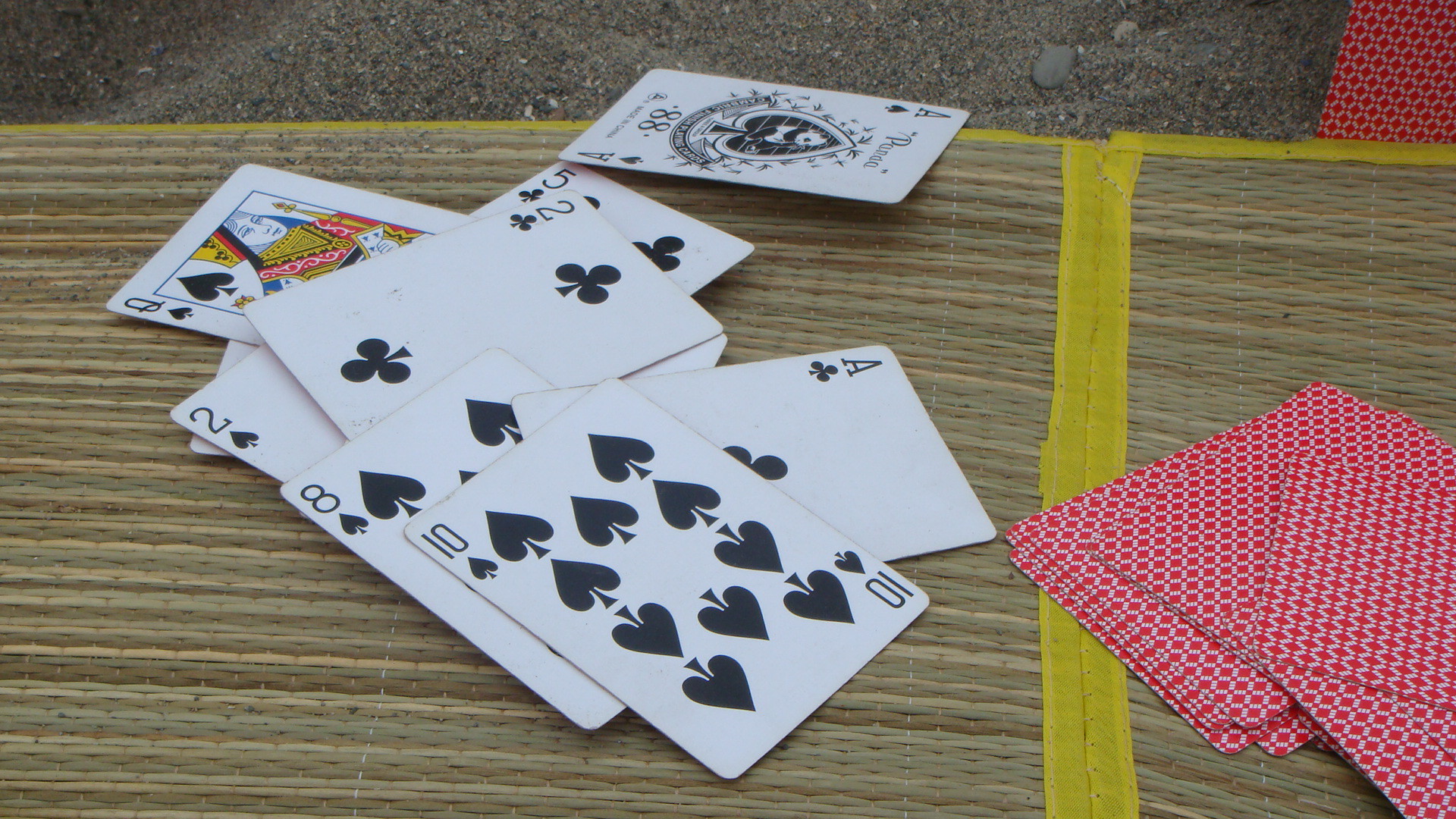A scattered deck of cards lies atop a grass straw mat with yellow-edged seams, positioned on a black pavement interspersed with small stones. The majority of the deck remains in a central pile, face down, while a few cards have slid to the side. Some cards are face up, specifically displaying black suits—spades and clubs—in no specific order. One card has even blown to the edge and rests face down on the ground. The scene is devoid of human presence, leaving an air of randomness and curiosity as to why the cards are arranged in this manner.